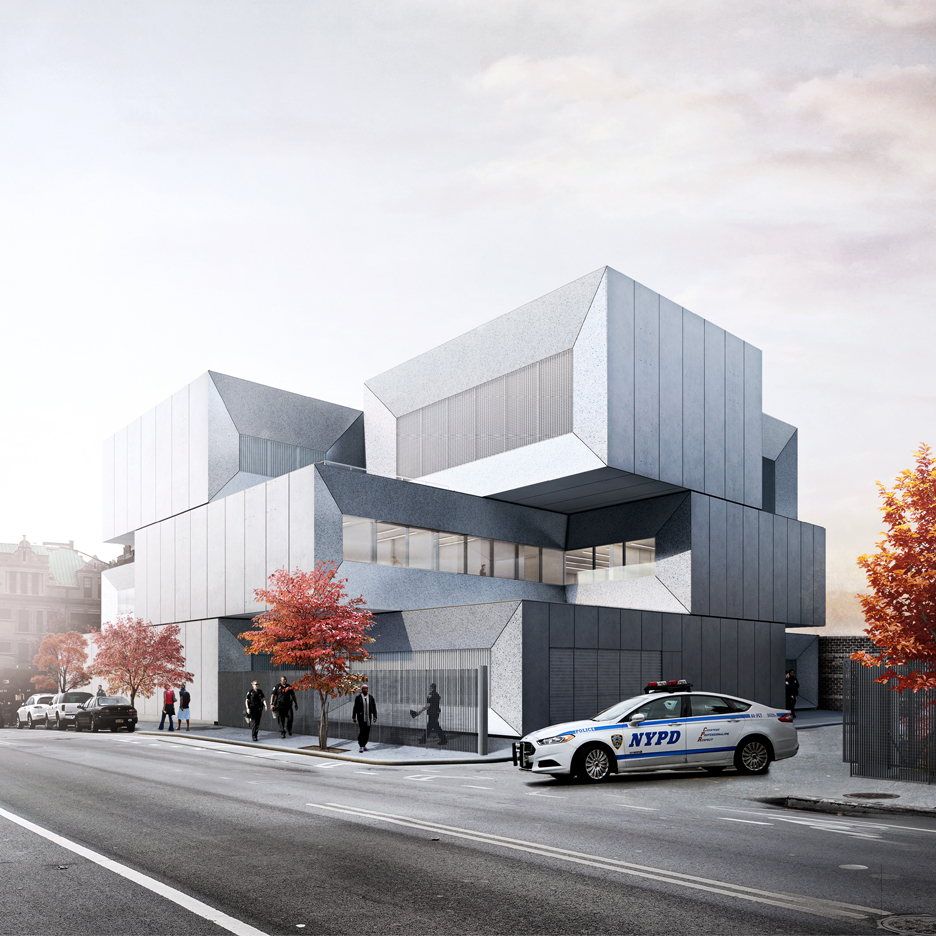This image is a highly detailed illustration, possibly a digital rendering or a still from a video game, showing a contemporary city street scene dominated by a large, modern building resembling stacked shipping containers or metal blocks. This three-story structure, which appears to be a police station, is predominantly gray with a strikingly boxy and futuristic design. The first and second floors have a few semi-transparent windows, adding to the building's sterile and geometric aesthetic. The scene is set against a gray sky with matching gray streets, emphasizing a monochromatic palette.

On the sidewalk in front of the building, five figures walk: two uniformed policemen, a man in a black suit, and two other pedestrians. A white NYPD police cruiser, marked by blue letters and seemingly ready to enter the street, is parked to the right of the building. The sidewalks are adorned with trees, both in front of the building and beside the police car, featuring reddish-orange leaves that inject a touch of color into the otherwise gray environment. In the background on the left, additional cars are parked along the street, adjacent to a large stone building with a light green roof, providing contrast and context to the urban setting.